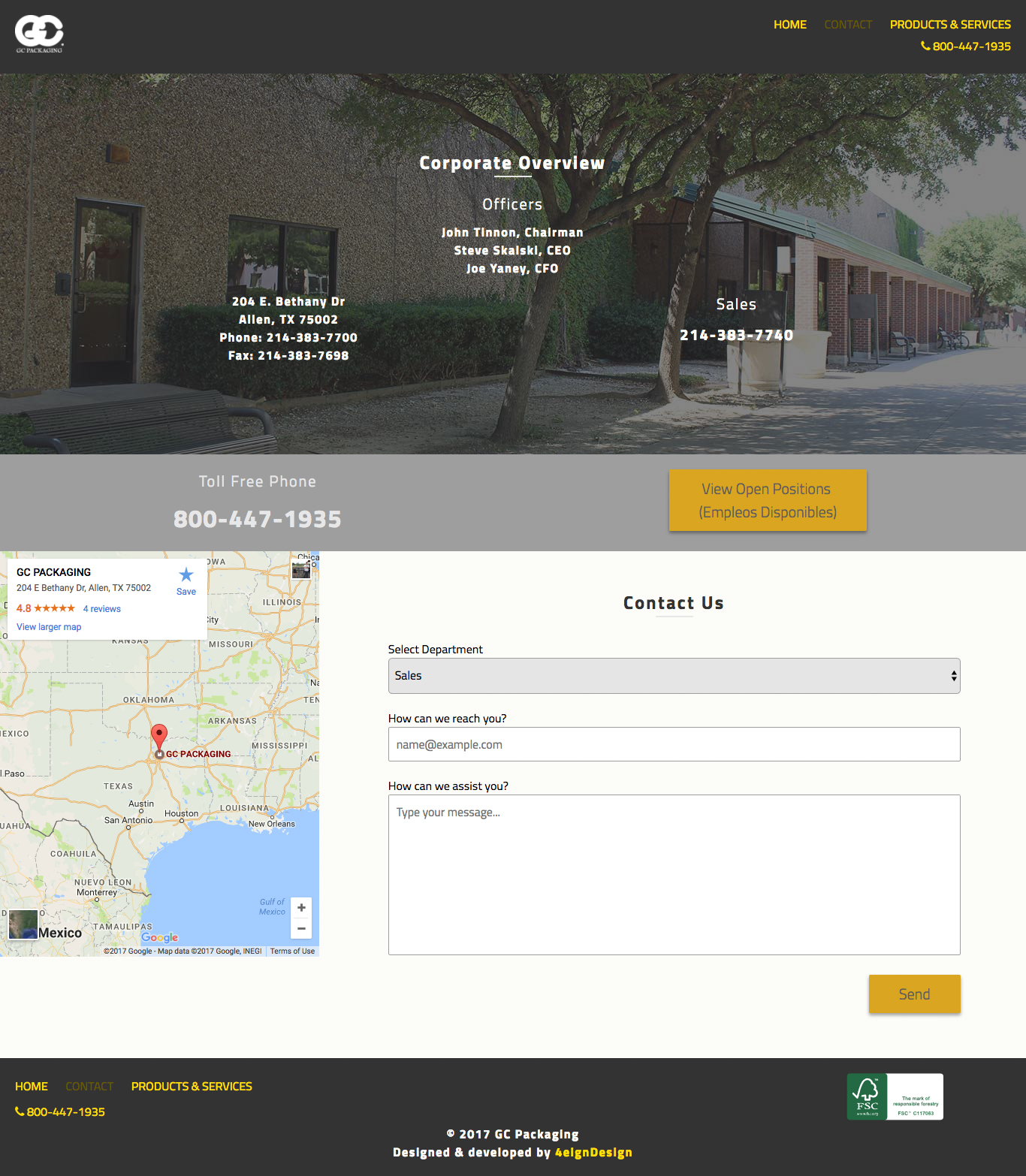**Caption:**

The website for GC Packaging features a prominent GC logo in the upper left-hand corner, composed of thick, interlocking letters resembling chain links. This logo is placed on a dark gray strip that runs across the top of the page. To the right of the logo, the menu options are listed in yellow text: Home, Contact (grayed out as it is the current page), and Protestant Services, with a phone icon and the number 800-447-1935 below.

On the Corporate Overview section of the Contact page, profiles of the company's executive officers are displayed, including John Tinnen, Chairman; Steve Skaliski, CEO; and Joe Yanni, CFO. To the left of these profiles, the company's address is provided: 204 East Bethany Drive, Allen, Texas, along with the zip code, phone, and fax numbers. A separate sales contact number, 214-383-7740, is listed on the right beside these details. Below this section, a gray line carries the toll-free phone number, 800-447-1935, in white, and a floating yellow button labeled "View Open Positions for Employee Disponibles."

Just beneath a banner, an inset Google map indicates the location of GC Packaging in Texas. The Contact area on the right side of the page allows users to select the Sales department (currently highlighted in gray), and provides fields to enter an email (placeholder: name@example.com) and a message. A yellow 'Send' button is available beneath this form.

At the bottom of the page, a gray footer repeats the menu options and phone number, includes copyright information, and features an FSC logo in the bottom right corner.